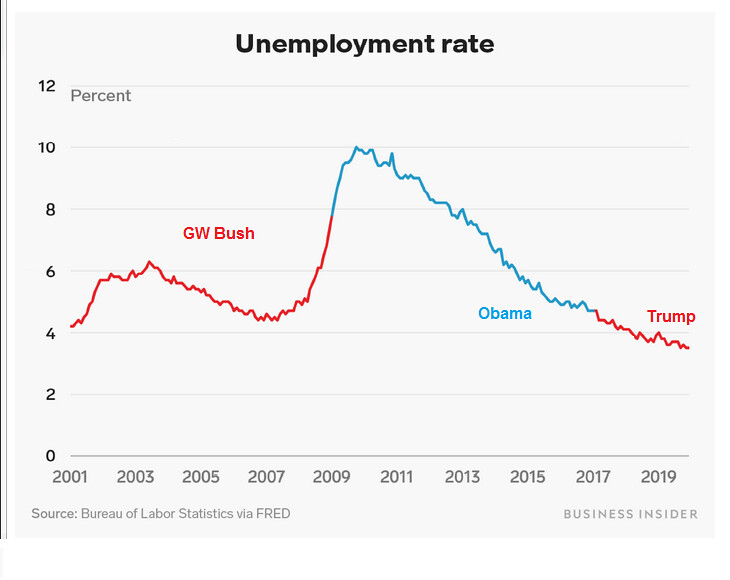The image displays a detailed line graph titled "Unemployment Rate" in bold black text, illustrating the unemployment trends from 2001 to 2019. The x-axis marks the years, while the y-axis represents the unemployment rates as percentages, ranging from 0 to 12%. The graph also distinguishes the tenures of three U.S. Presidents, using different colors: George W. Bush's tenure (2001-2009) is marked in red, Barack Obama's tenure (2009-2017) in light blue, and Donald Trump's tenure (2017-2019) in a reddish hue.

In 2001, the unemployment rate began just above 4%, rising to around 6% by 2003 during George W. Bush's presidency. The rate then briefly declined to approximately 5% by 2007 before climbing steeply to nearly 8% in 2008. Under Barack Obama, the unemployment rate peaked at around 10% in 2010 but gradually decreased to approximately 4.5% by the end of his tenure in 2017. During Donald Trump's term, the unemployment rate continued to decline, ending slightly below 4% by 2019. The graph vividly captures the fluctuating unemployment rates across these presidential terms and highlights significant economic shifts over the years.